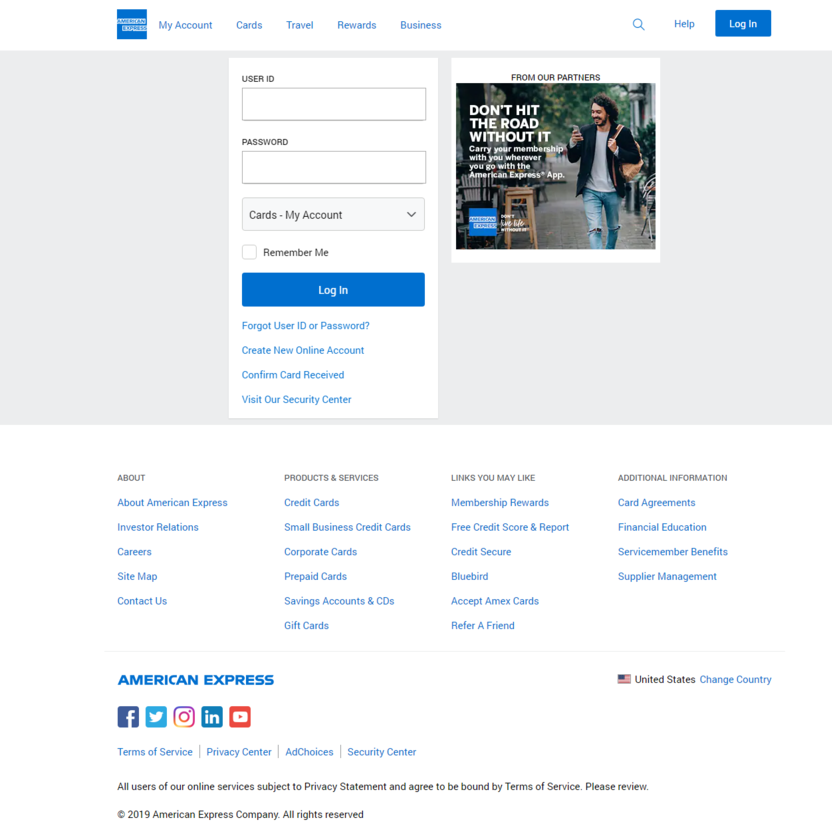This detailed screenshot of the American Express webpage showcases the layout and key features prominently. At the top, the menubar displays navigation options including My Account, Cards, Travel, Rewards, and Business, aligned in a row next to the American Express logo. The main body of the homepage features two distinct sections:

On the left, there's a login box where users can enter their User ID and Password. The login form includes a drop-down menu labeled 'Card My Account' and a 'Remember Me' checkbox for user convenience. Beneath these, a prominent blue 'Login' button stands out. Below the login button, four helpful links are present: 'Forgot User ID or Password,' 'Create New Online Accounts,' 'Confirm Card Reviews,' and 'Visit Our Security Center.'

The right side of the page displays an advertisement from an American Express partner. The ad encourages users to carry their membership with them by using the American Express app, under the tagline "Don't hit the road without it."

At the bottom, the footer is divided into four sections: About, Products and Services, Links You May Like, and Additional Information. In the lower left corner, the footer features the American Express logo in blue and all caps, alongside icons for popular social media platforms including Facebook, Twitter, Instagram, LinkedIn, and YouTube.